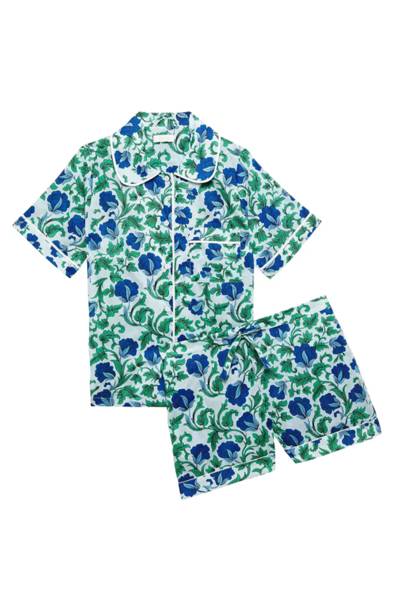The photograph depicts a matching set of apparel laid out on a white background, resembling a product thumbnail typically seen on an e-commerce website. The set consists of a short-sleeved collared shirt and a pair of shorts, both adorned with a vibrant floral pattern featuring blue flowers and green leaves. The shirt includes a pocket and a rounded, thick collar. The shorts are styled to about thigh level with rolled-up bottoms and are positioned at a counterclockwise angle, slightly overlapping the shirt. Both items showcase the same print, suggesting they are either pajamas or a casual summer set, potentially designed for men. The white background accentuates the detailed and lush floral design, emphasizing the seamless coordination between the shirt and shorts.